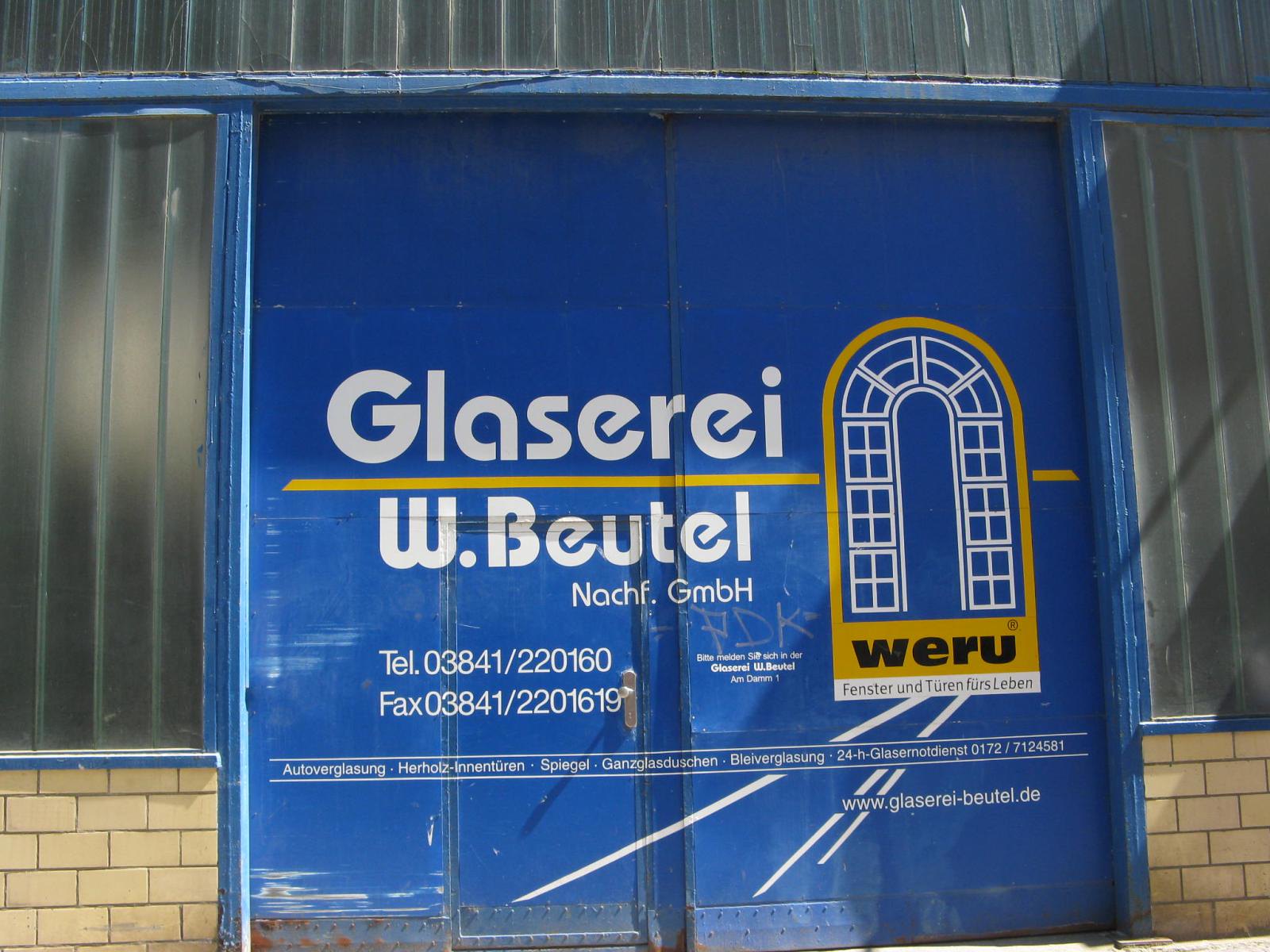The image depicts a large blue sliding door framed by vertical glass panels with opaque material. The door is part of a building that has a light yellow brick wall at the bottom, supporting the glass panes. The blue door features prominent white text that reads "GLASEREI" at the top. Below this, a horizontal yellow line separates the upper text from "W. BEUTEL." Further down in smaller white lettering is "NACHF. GMBH," followed by a telephone number "TEL. 03841/220160" and a fax number "FAX 03841/2201619."

On the right half of the door is a U-shaped, upside-down arch logo outlined in yellow, resembling a decorative window you'd find in a mansion. Below this logo, the word "WERU" is displayed in black letters on a golden outline. A horizontal rectangular bar with black lettering too small to read is situated beneath this. Towards the bottom, two small white horizontal lines enclose additional unreadable text.

Above the doors are additional glass sections that may be metal-framed. These elements give a complete view of an old building facade with a modern sign and contact details prominently displayed.